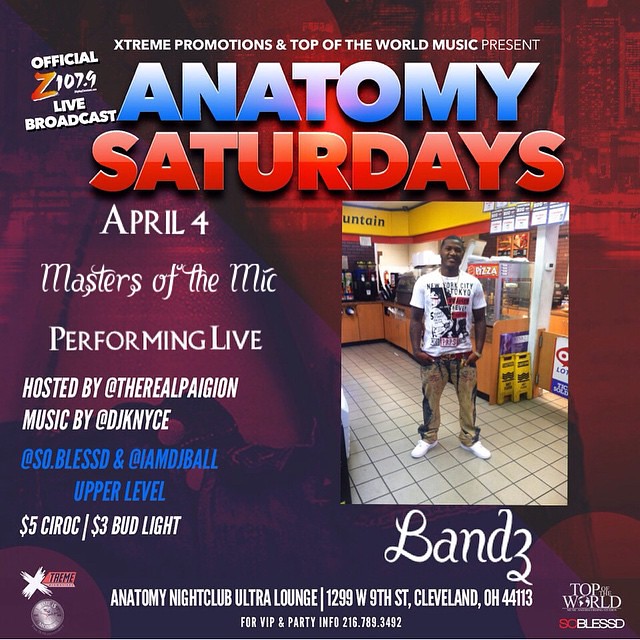**Event Flyer Description:**

At the top of this striking flyer, bold text declares "Extreme Promotions and Top of the World Music Present: Anatomy Saturdays." 

In the upper left-hand corner, an eye-catching note announces an "Official Z 107.9 Live Broadcast."

Centered prominently on the flyer, details of the main event are highlighted: 
- "April 4th Masters of the Mic Performing Live"
- Hosted by The Real Pagion
- Music by DJ K Nice

Further down, additional entertainment is specified:
- "So Blessed" and "I Am DJ Ball Upper Level"

A tempting note follows, promoting special drink offers:
- "$5 Ciroc"
- "$3 Bud Light"

To the right side of the flyer, a vibrant photograph captures a young Black man standing inside a convenience store. He is stylishly dressed in a white t-shirt featuring black and red print, paired with dark denim jeans and white sneakers. Below the image, the text "Band 3" is displayed.

At the bottom, the venue information is provided:
- "Anatomy Nightclub Ultra Lounge"
- "1299 West 9th Street, Cleveland, Ohio"
- For VIP and party info, a contact phone number is given.

This well-designed flyer promises an electrifying evening filled with live performances, fantastic music, and unbeatable drink specials at a premiere nightlife destination.